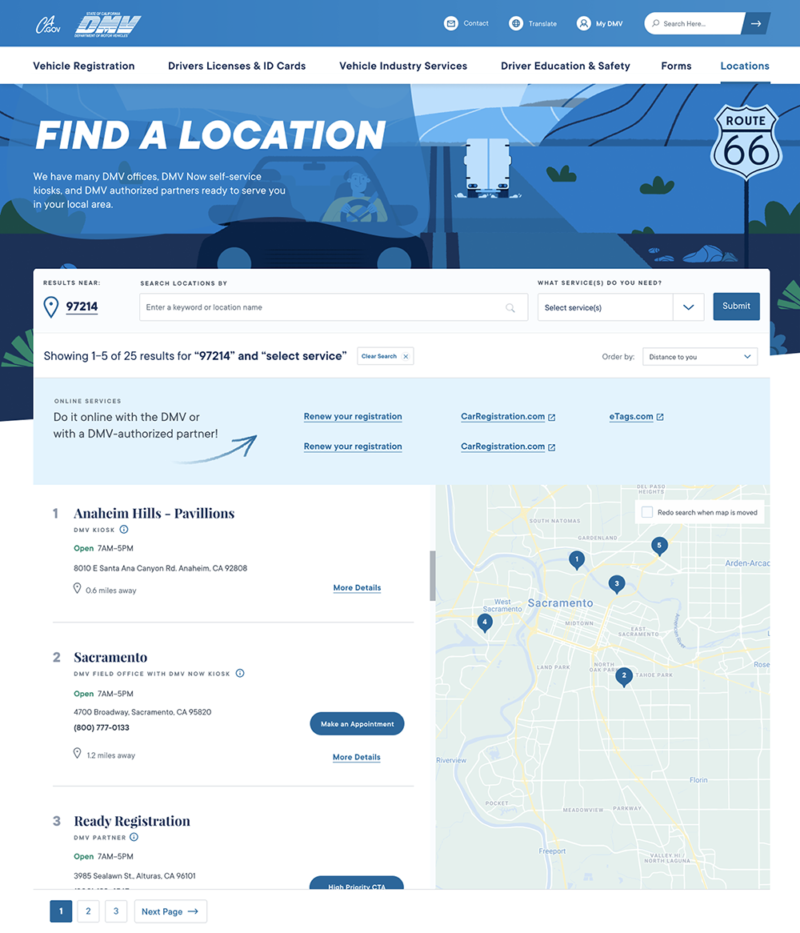**California DMV Location Finder Webpage**

The webpage for the California Department of Motor Vehicles (DMV) focuses on assisting users in finding a DMV location near them. The California DMV (CADMV) logo is prominently displayed. Small icons for Contact, Translate, and MyDMV with a Login option provide quick access to essential services. The navigation menu includes options for Vehicle Registration, Driver's License, ID Cards, Vehicle Industry Services, Driver Education and Safety, Forms, and Locations.

A clear heading states, "Find a Location." The page highlights various service points, including many DMV offices, DMV Now self-service kiosks, and DMV-authorized partners available in your local area.

The background image features an illustration of a person driving a car down Route 66, surrounded by historic road signs.

The central search section allows users to search for locations by inputting a zip code, in this example, 97214. Users can also search by keyword or location name, select services from a dropdown menu, and click the search button. The search results, which display 1 through 5 out of 25 results for zip code 97214, provide detailed information about each location.

**Search Results:**

1. **Anaheim Hills Pavilion**
   - **Status:** Open from 7 a.m. to 5 p.m.
   - **Address:** 8016 East Santa Ana Canyon Road, Anaheim, California, 92808
   - **Distance:** 0.6 miles away

2. **Sacramento**
   - **Status:** Open from 7 a.m. to 5 p.m.
   - **Address:** 4700 Broadway, Sacramento, California, 95820
   - **Phone Number:** 800-777-0133
   - **Distance:** 12 miles away
   - **Additional Information:** Link to make an appointment and more details

3. **Ready Registration**
   - **Status:** Open from 7 a.m. to 5 p.m.
   - **Address:** 3985 Seawall Street, Alturas, California, 96101
   - **Additional Information:** High priority GTA link

Additionally, the page offers links to renew registration online via DMV authorized partners like CarRegistration and eTags.com. Navigation at the bottom of the page allows users to go to subsequent pages (page 2, page 3, etc.).

A map on the webpage pins the locations of the DMVs corresponding to the listings, ensuring a visual guide for users. The website boasts a clean, professional design with an intuitive and user-friendly interface, making it easy for users to navigate and find the services they need.